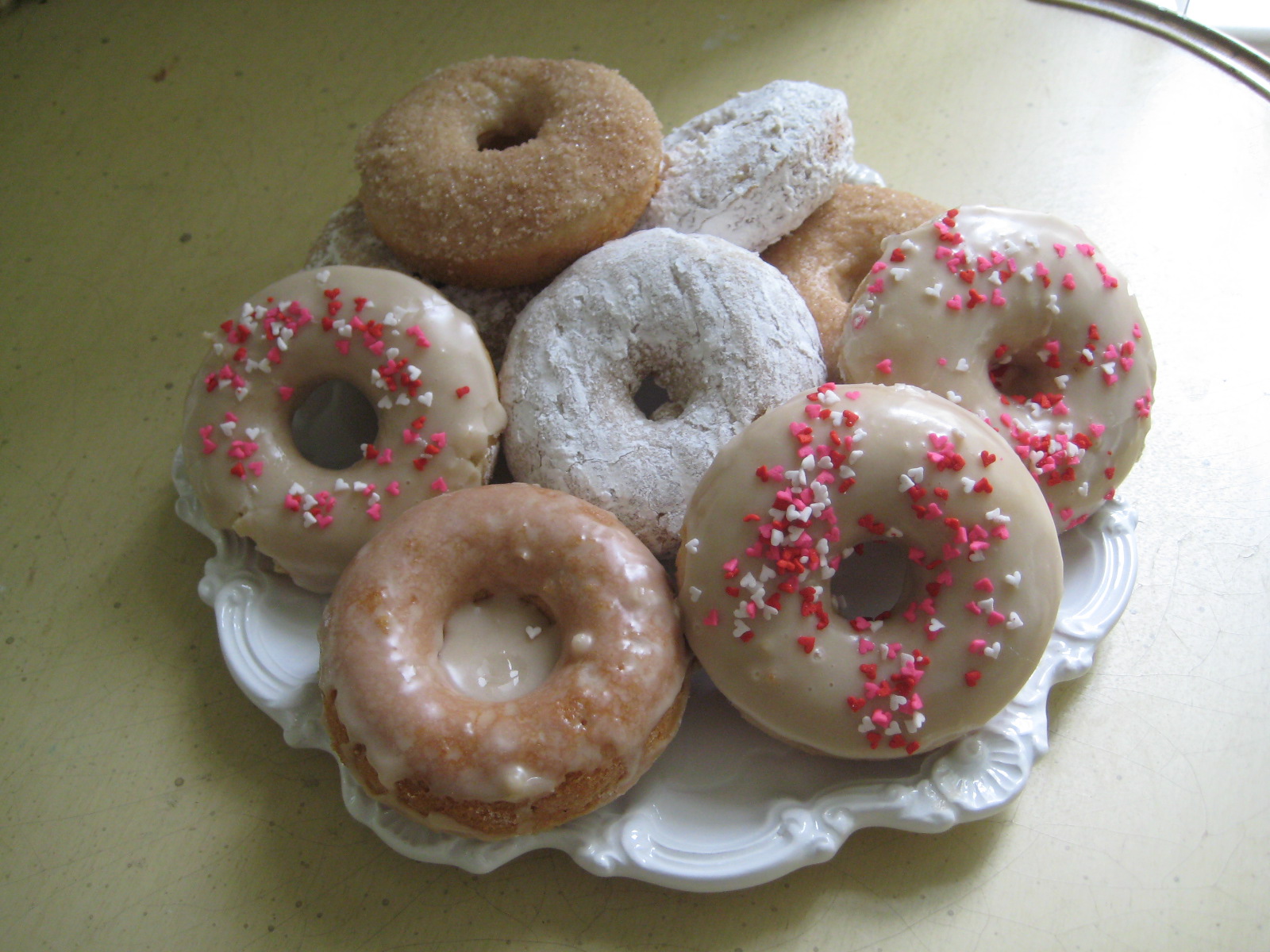This detailed color photo showcases a collection of nine assorted doughnuts artfully arranged on a white ceramic plate with scalloped, floral scroll-patterned edges. The plate casts a slight shadow on the light tan tabletop below. The doughnuts, varying in types and toppings, include: plain glazed doughnuts, doughnuts dusted with granulated and powdered sugar, and doughnuts adorned with a light tan icing sprinkled with pink, white, and red heart-shaped sprinkles. The stack of doughnuts, some of which appear to be cake doughnuts, is rich and tempting, though clearly indulgent. The table, illuminated by streaming light, adds a warm ambiance to the setting, though it appears slightly unclean in places, enhancing the photo’s casual, everyday charm.